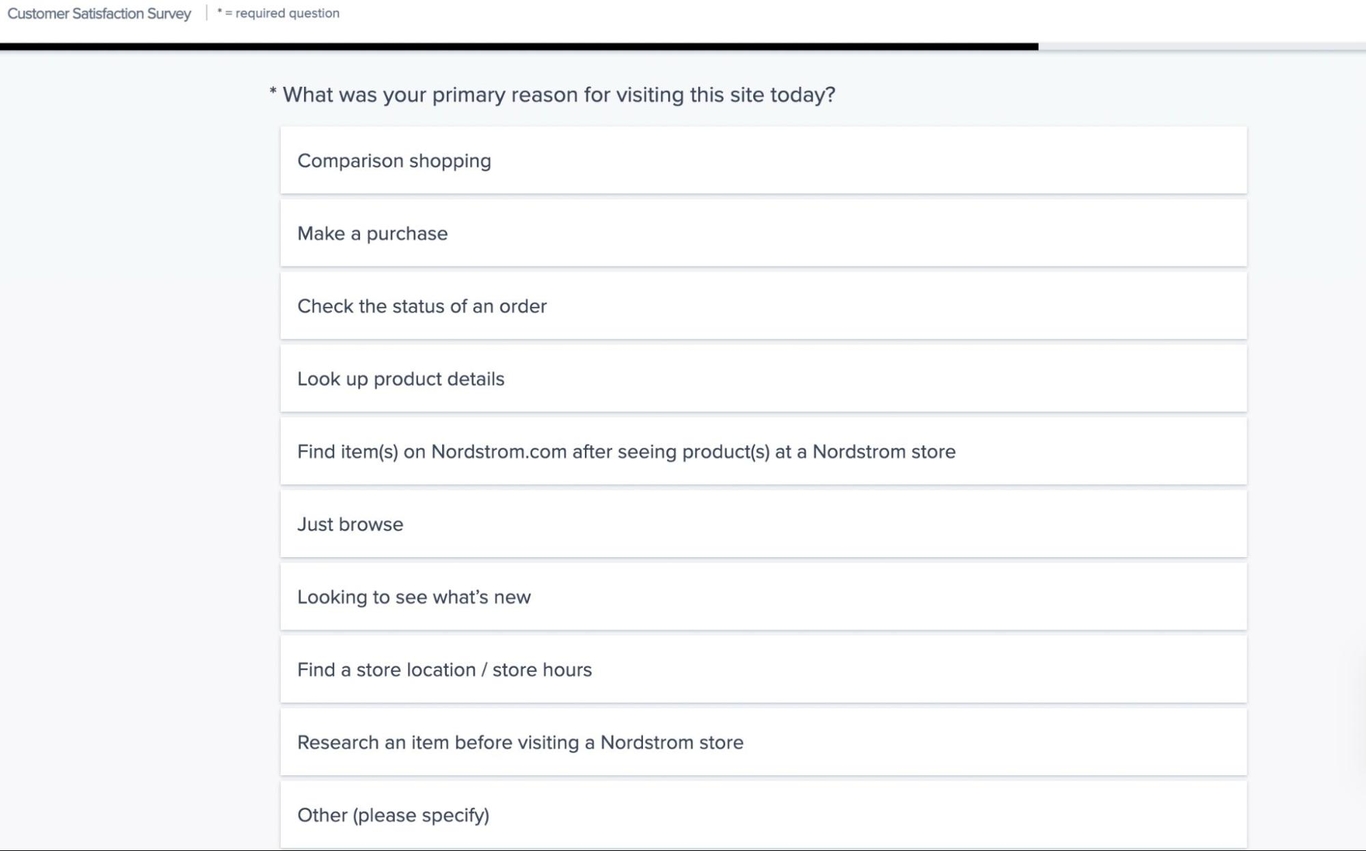The image depicts a webpage designed for a customer satisfaction survey. The webpage has a clean, minimalist design with a white background and black text. At the top of the page, the title "Customer Satisfaction Survey" is prominently displayed in black font, accompanied by an asterisk indicating that certain questions are required. Below the title, a status bar spans the width of the webpage, predominantly black with a segment that is white, possibly indicating user progress through the survey.

Beneath the status bar, the survey poses a key question in bold text: "What is your primary reason for visiting this site today?" To facilitate responses, several rectangular option boxes are listed, each containing different selectable reasons for visiting the site. The options include:

1. Comparison shopping.
2. Make a purchase.
3. Check the status of an order.
4. Look up product details.
5. Find items on Nordstrom.com after seeing products at a Nordstrom store.
6. Just browse.
7. Looking to see what's new.
8. Find a location/store hours.
9. Research an item before visiting a Nordstrom store.
10. Other (with a prompt to specify).

Each option is clearly delineated for the user to select their specific reason for visiting, indicating a well-organized and user-friendly survey interface.